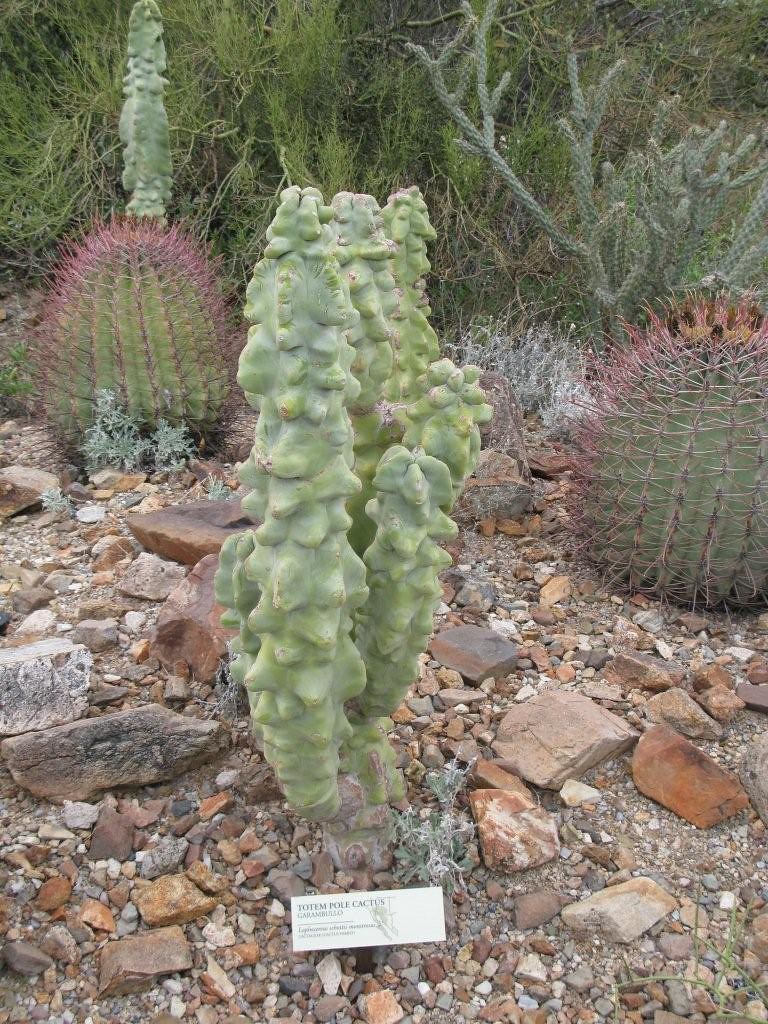This outdoor photo features a rocky terrain adorned with various types of cacti. Dominating the center is a tall, pale green Totem Pole Cactus, characterized by its bumpy surface and multiple upright branches, around four to six in total. Smaller buds are seen on the right side, with one particularly tiny one on the left. At the base of this central cactus is a white rectangular card with black lettering that reads "Totem Pole Cactus." Flanking this central cactus are traditional, almost perfectly round green cacti with reddish-brown spikes—one on each side of the photo. Behind the round cactus on the left, another Totem Pole Cactus peers out. Additionally, behind the round cactus on the right, there is a different species of cactus with numerous thin, antler-like branches. The ground is a mix of small and large rocks, adding to the desert-like ambiance, while some greenery can be faintly observed in the very background.